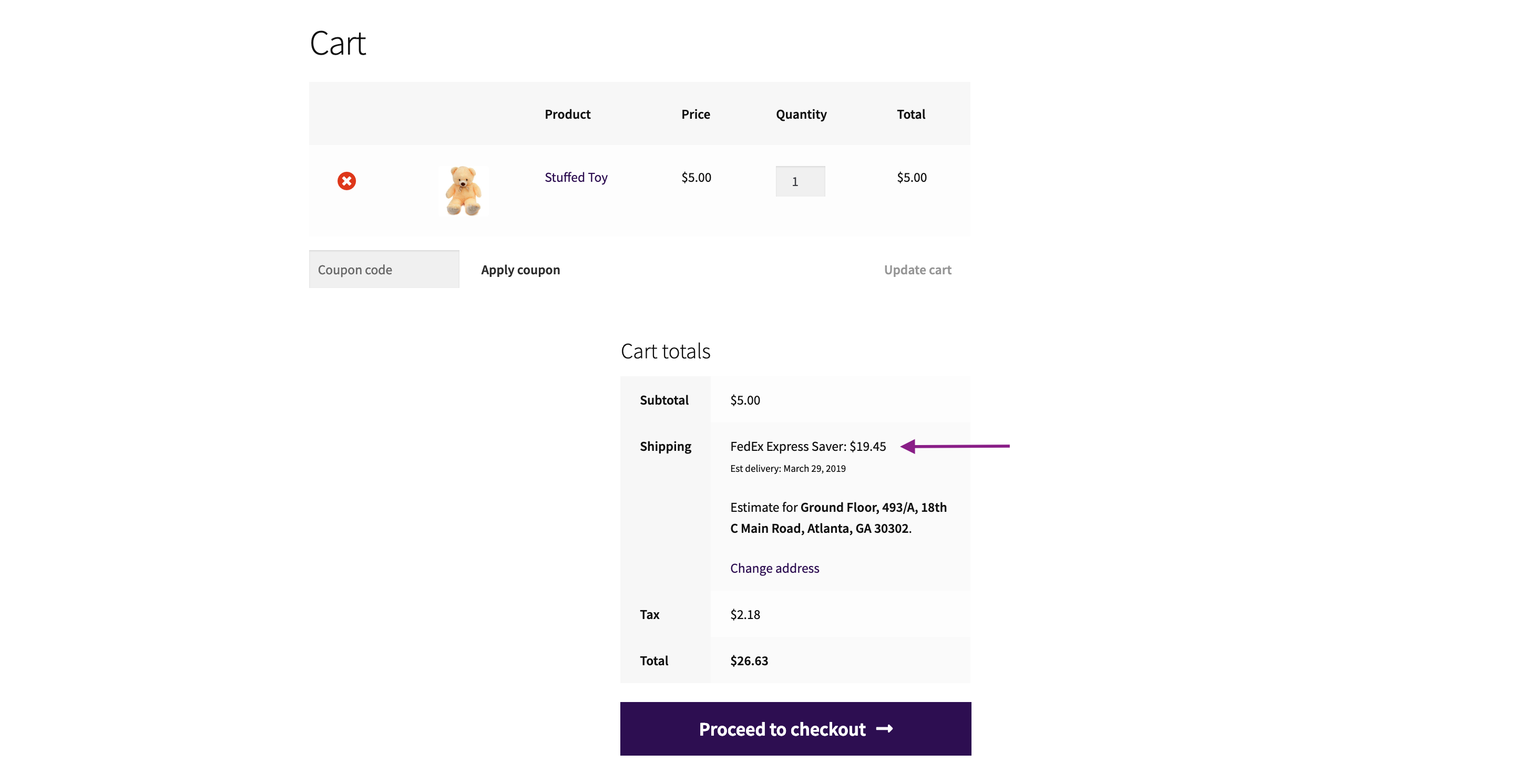The web page displays a predominantly white background with sections of varying shades of gray. In the top left corner, "CART" is prominently displayed. Just below, a light gray rectangle with a darker hue features dark blue or purple text organized in a table format with headings: "Product," "Price," "Quantity," and "Total."

In a subsection characterized by lighter gray, a red circle with a white 'X' icon is seen. Adjacent to this icon is an image of a light tan teddy bear with orange accents and feet that appear either gray or dark tan. The product description reads "Stuffed Toy," priced at $5. The quantity is specified as 1 within a dark gray rectangle, and the total cost is also $5. Below this, there is a section for a coupon code, displayed in dark gray, with an "Apply Coupon" button in bold black. To its right, "Update Cart" is indicated in gray.

Further down, the page displays "Cart Totals" in black font. A section labeled "Subtotal" in blue indicates a cost of $5. The shipping method is specified as "FedEx Express Saver" at a cost of $19.45, highlighted by a purple arrow pointing at it. The estimated delivery date is March 29, 2019. Under this, the delivery address is specified with the following details in bold:  
"Ground Floor, 493/A, 18th C Main Floor Road, Atlanta, GA 30302."

The user is prompted to "Change Address" below this detail. Tax is listed as $218, bringing the total to $2663. At the bottom, there is a dark blue button with bold white text stating "Proceed to Checkout," accompanied by an arrow pointing to the right.